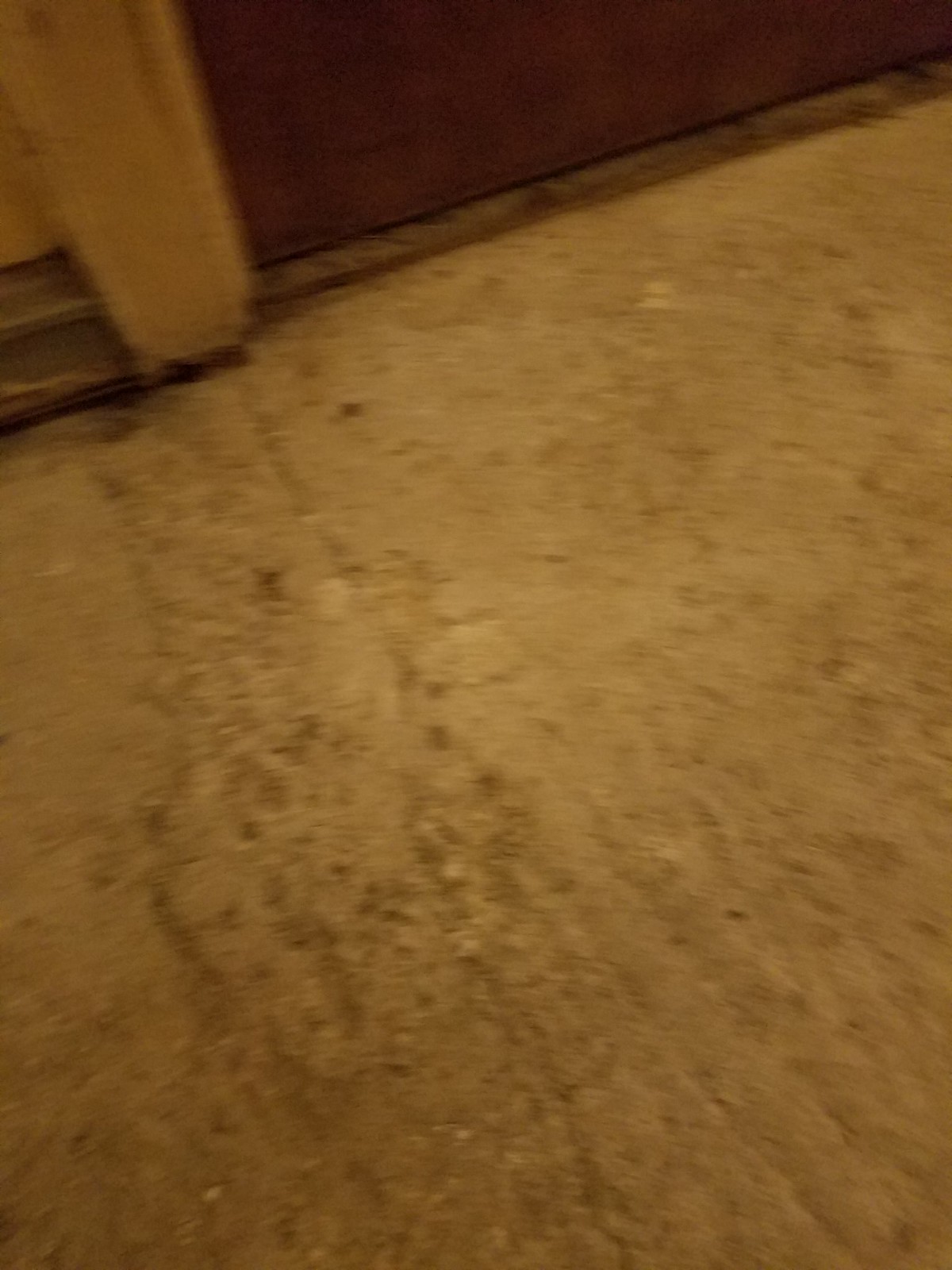In this image, we see a poorly taken, blurry photo in portrait orientation, capturing what appears to be an outdoor area with a dirt or sand-like, light brown floor, marked by cracks. Off to the left, there is a two-step dark gray concrete slab ascending, possibly leading to a yellow door, though the door is not entirely visible. Adjacent to this, an orange column stands upright, possibly on a cement base, reaching upward. A brown wall, situated on grayish concrete, is also partly visible to the left of the column. The photo looks like it was taken from a downward, diagonal angle, as if snapped by accident, with no distinct subject, making it somewhat disorienting.